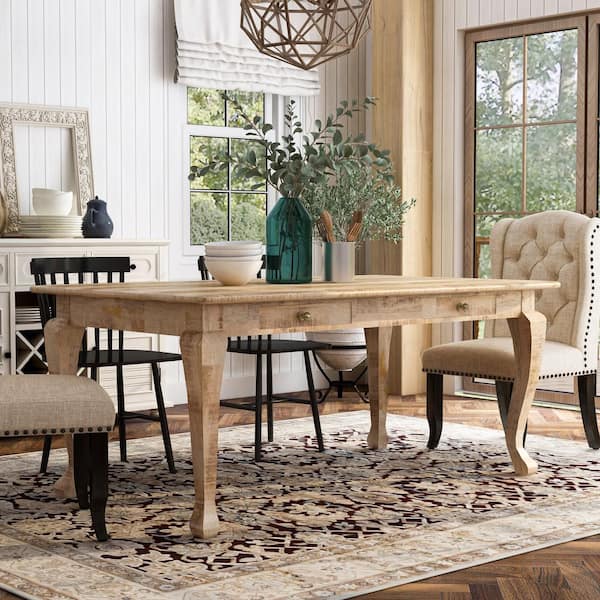The image depicts a modern yet minimalistic countryside dining room featuring a light oak dining table with thick legs atop an ornate rug, blending white, black, and brown hues, on a hardwood floor. The table is surrounded by four chairs: two black wooden ones on the sides and two plush, white upholstered armchairs at each end, noted for their comfort and metal beading details. The table is minimally decorated with a green vase holding fake eucalyptus plants and some white ceramic bowls. The dining room walls are painted white wood, enhancing the airy feel of the space. Behind the dining table, there's an end table stocked with various plates, bowls, and a teapot, suggesting a ready-to-use dining setup. The room is well-lit by a lamp overhead and natural light streaming in through two windows, which offer a view of a nearby wooded area.